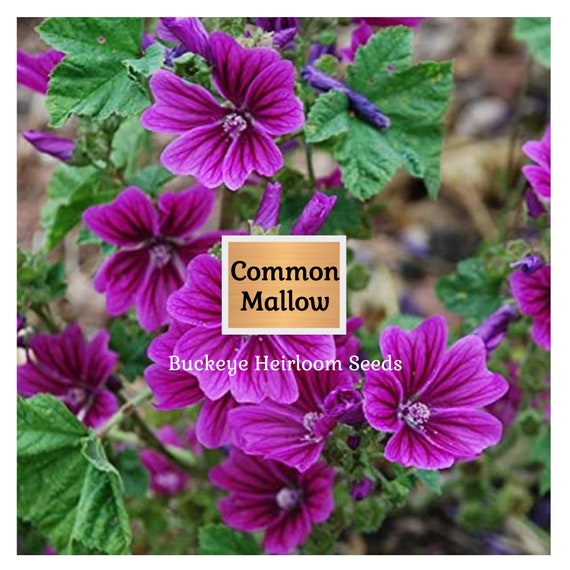The advertisement for Buckeye Heirloom Seeds showcases a stunning close-up photo of vibrant Common Mallow flowers. These deep purple or magenta blooms, veined with rich hues, contrast beautifully against lush green leaves. The plant is teeming with numerous blossoms, adding to its lush and abundant appearance. Right at the center of the image, a tasteful label features the flower's name, "Common Mallow," in an elegant curly font set against a brown woody background, framed in white. Below this, the company name "Buckeye Heirloom Seeds" is prominently displayed in matching curly black lettering, harmonizing with the rustic aesthetic. This well-composed photograph captures the eye-catching beauty and vibrancy of the Common Mallow, making it an ideal advertisement for the garden seed company.